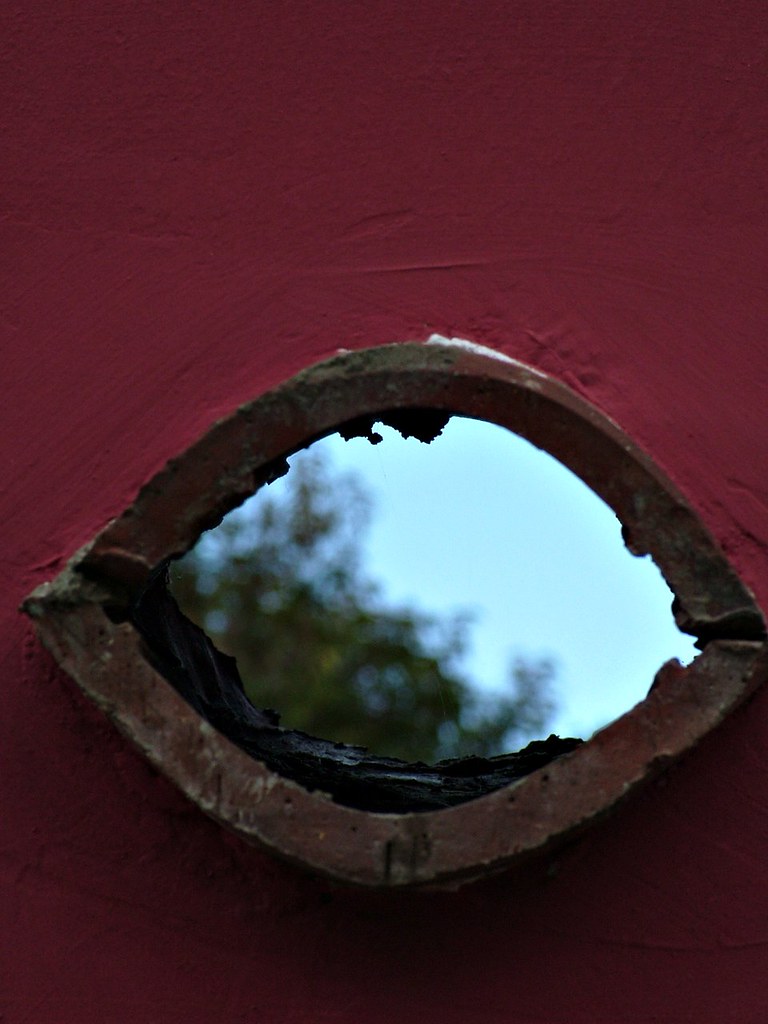A striking image captures a section of a vibrant red wall with a large, circular break. The rough edges of the break are rusted and worn, adding texture to the scene. Through the jagged aperture, a clear blue sky is visible, framed by the lush green leaves of a tree, creating a stark yet captivating contrast between the man-made structure and the natural world beyond.